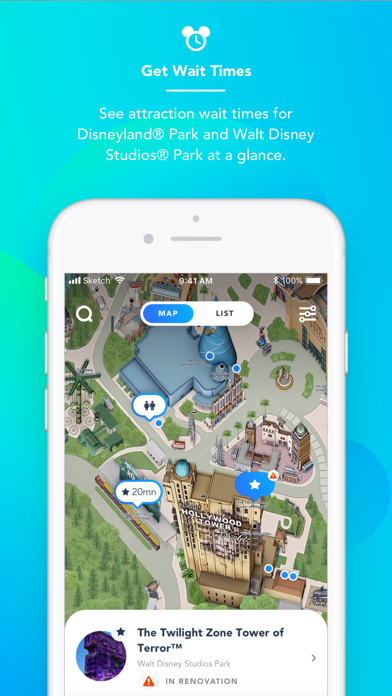This descriptive caption provides a detailed overview of the Disneyland app's screenshot:

"In the screenshot of the Disneyland app, the header displays a teal background featuring the text 'Get Wait Times' prominently at the top. Accompanying the text is an icon of Mickey Mouse ears with a clock inside, symbolizing the wait times feature. Below this header, a description in teal text reads, 'See attraction wait times for Disneyland Park and Walt Disney Studios Park at a glance.' Central to the screenshot is an image of an iPhone with a white bezel, showing the app's interface. The screen depicts Disneyland attractions, with the iconic Hollywood Tower and other park buildings prominently displayed. At the top of the app interface, options for 'Map' and 'List' views are visible, along with typical iPhone system icons including Wi-Fi signal, 4G status, time, and battery level. At the bottom of the app screen, detailed information about the Twilight Zone Tower of Terror indicates that the attraction is 'In Renovation.' The iPhone's bezel also displays physical buttons for power and volume control along its side."